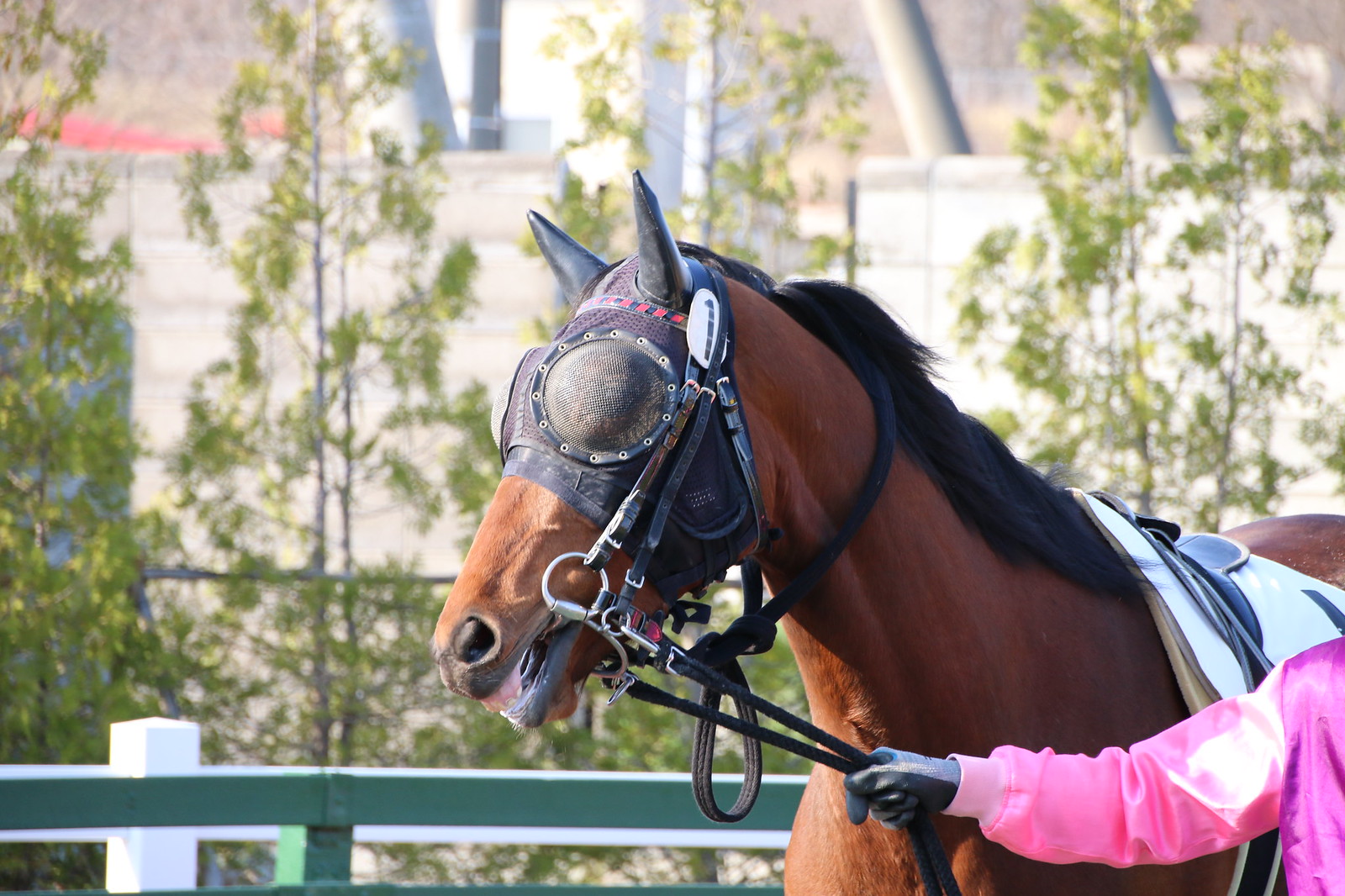This is a vibrant color photograph taken outdoors on a bright, sunny day, showcasing a landscape orientation. A dark brown horse with a black mane is being led by a trainer in the foreground. The trainer, visible by her arm and shoulder, sports a pink jacket and black gloves. The horse, fitted with blinders that cover its eyes and ears, is also saddled, suggesting it might be ridden later.

Behind the duo, a green and white wooden fence runs parallel to their path. Further back, scraggly, leaf-budding trees, likely in early spring, punctuate the scene. Interspersed among the trees are some industrial-looking structures and metal rods, adding an intriguing contrast to the natural setting.